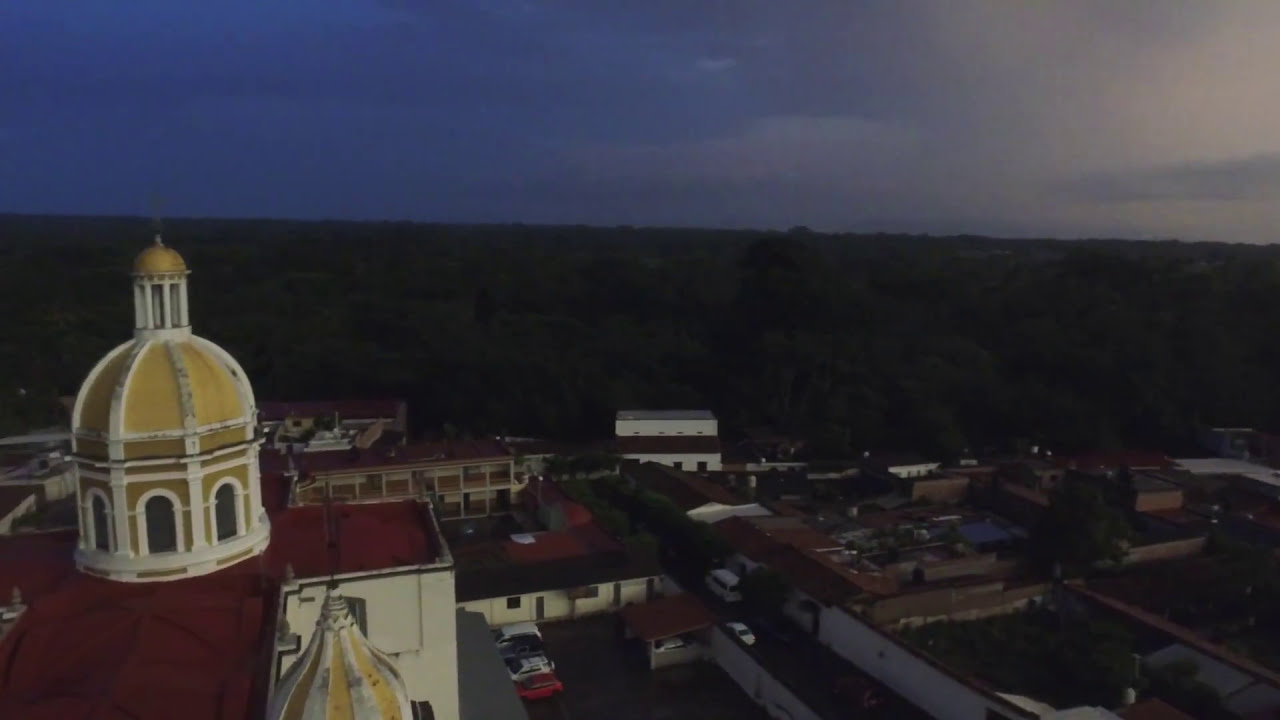This aerial image, likely captured by a drone, showcases a picturesque small village that appears to be set in a non-American, possibly Indian, locale. Dominating the lower left corner of the frame is a striking white building with a red roof, adorned with two yellow domes accented with white trim—resembling a church or cathedral. This unique structure stands out amidst an assortment of smaller, flat-roofed buildings and enclosed spaces defined by fences. In the lower part of the image, cars are visible on a grey road and in parking lots, possibly affiliated with the domed building. Surrounding the village is a dense, dark green forest that stretches to the horizon. The sky above transitions from a clear blue on the left to more overcast conditions on the right, with sunlight breaking through the clouds, suggesting the photo was taken either in the early morning or late evening.